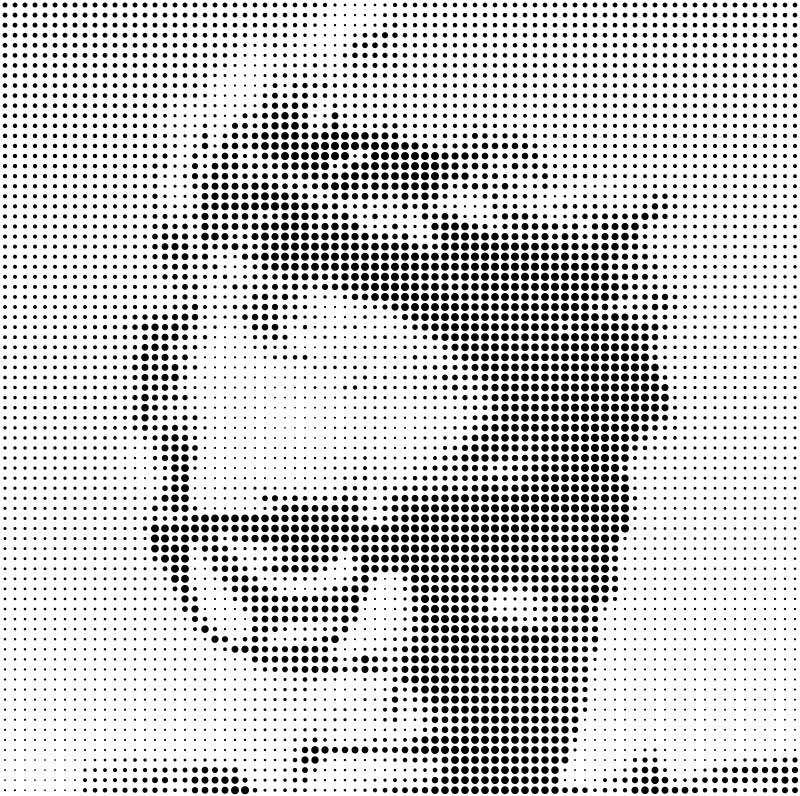The image depicts an androgynous person with very short, disheveled hair, wearing thick, black-framed glasses. The entire visual is composed of dots varying in size—larger and denser where the shadows are darker, and smaller and sparser where the light areas emerge, giving it an artistic, print-like quality. The person’s facial features are faintly outlined; you can discern the outline of the eyes, nose, and a mouth that is set in a neutral expression, with the gaze directed straight ahead. It gives the impression of being a manipulated or computer-generated image, focused and zoomed in to the point that it omits the person’s chin and any background context. The intricate dot arrangement requires a trained eye to fully appreciate the portrait, as the image comes into sharper focus when viewed from a slight distance.